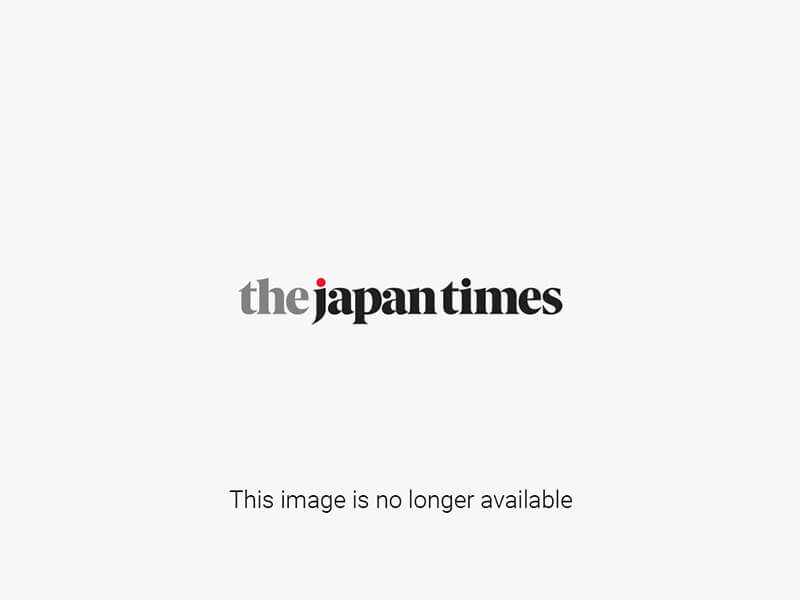This overhead image depicts a coastal area with a distinct contrast between deep, dark blue water on the left side and shallower, green-hued water on the right, indicative of a drop-off. There are approximately five boats or shipwrecks scattered in the deep blue section of the water. A specific area on the land is highlighted with a white, slightly curved box, though it remains pixelated and unclear. The shoreline itself appears rocky and varied in color, featuring greens, tans, and browns. Logos for CSIS, AMTI, and Maxar Technologies are displayed along the bottom right corner of the image.